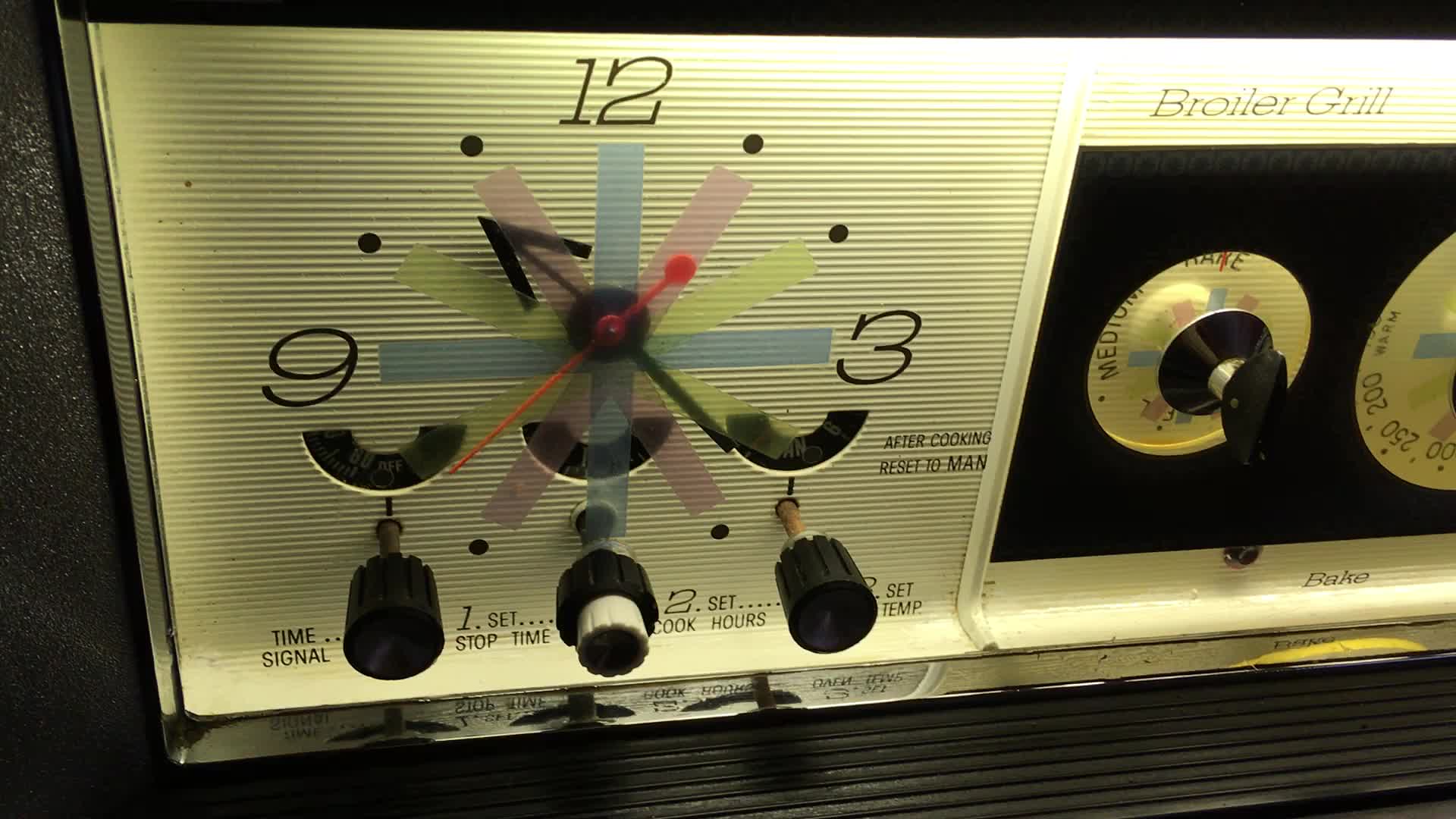The image features a vintage cooking appliance, partially visible, with a distinctive gold-colored front panel. On the left side of the front panel, there is a clock or timer display with a standard circular arrangement: 12 at the top, 3 on the right, 6 at the bottom, and 9 on the left. The clock includes various adjustment buttons positioned along the bottom, designated for setting the time, signaling alarms, and configuring other timing functions.

Adjacent to the clock on the right side, there is lettering that reads "Broiler Grill," indicating cooking modes. Below this, there is a dial with multiple settings, including "Medium Bake" and other temperature options marked in Fahrenheit. This suggests the appliance has multifaceted cooking capabilities. Despite the absence of clear manufacturer branding, the detailed settings and gold finish highlight its classic, functional design.